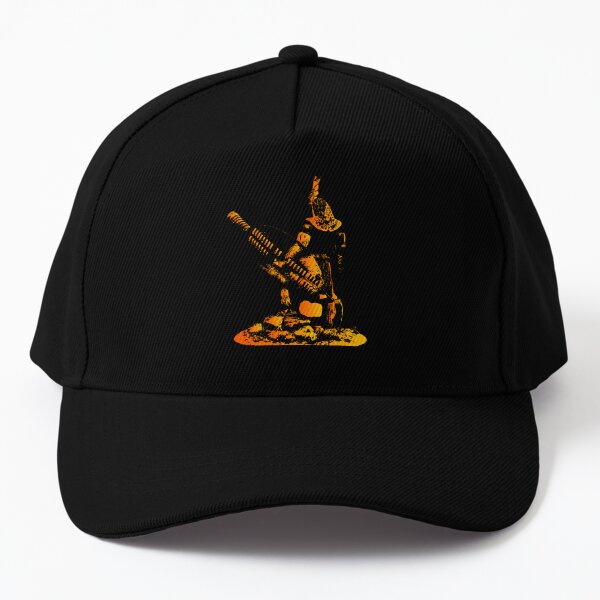This photograph showcases a simple yet detailed black baseball cap made from black fabric, viewed from the front. The cap features a slightly curved visor and the characteristic black button at the top. Prominently displayed in yellow embroidery on the front is a stylized figure standing on a pile of rocks. The figure, dressed in what appears to be traditional attire, could be interpreted in multiple ways: one viewer describes it as a man in a hat with a feather, possibly holding an instrument; another suggests it resembles a gladiator from behind, while a third observer speculates it might be a samurai kneeling, holding two swords in their scabbards, contributing to an Asian-inspired aesthetic. The yellow embroidery contrasts sharply with the black fabric, making the intricate design stand out despite its ambiguity. There is no text on the cap, emphasizing the unique and interpretive nature of the embroidered figure.